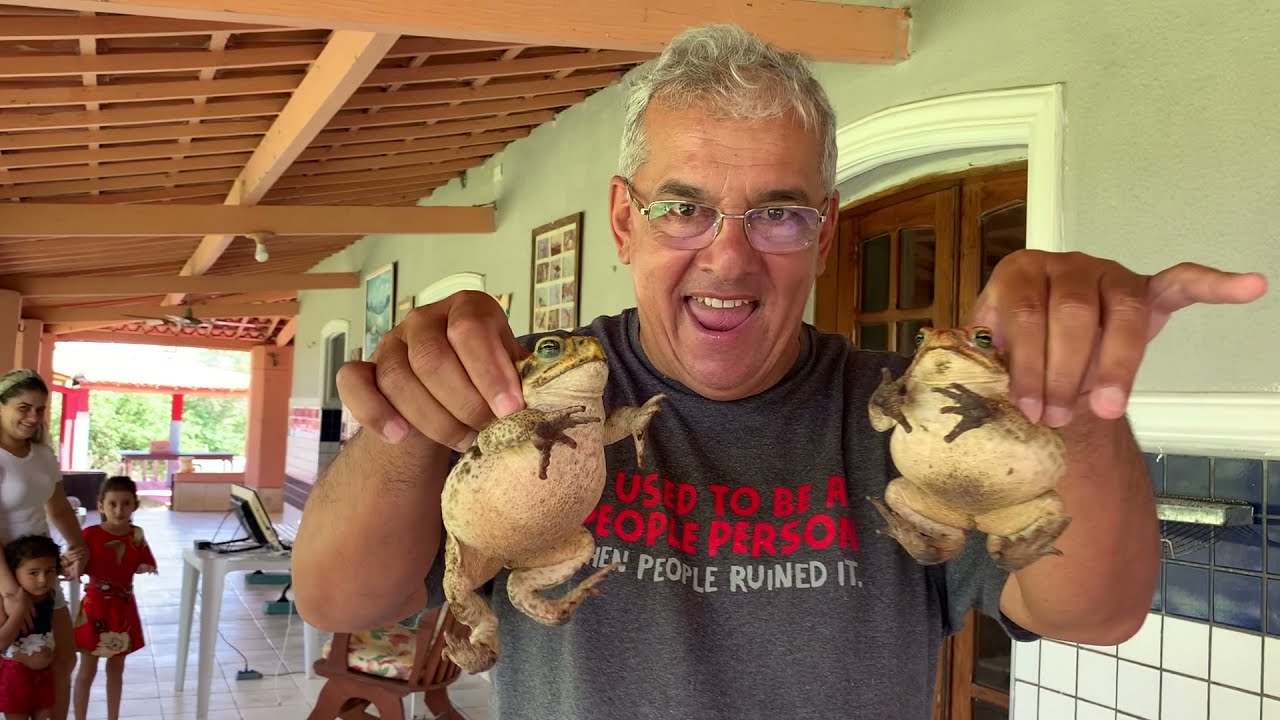The image captures a middle-aged man with short, slightly receding, curly gray hair, who is smiling with a slightly mischievous or sinister look on his face. He is wearing white-rimmed glasses and a dark gray t-shirt that reads "I used to be a people person" in red text and "then people ruined it" in white text. The man is centrally positioned but slightly to the right. He holds two frogs by their necks, one in each hand, with their bellies facing towards the camera. The frog in his left hand has its legs hanging down and arms outstretched, while the frog in his right hand appears more balled up with limbs close to its body. Both frogs have white undersides and green heads with light blue eyes. The setting is an outdoor area under a building's awning, featuring a background of white walls adorned with pictures and a brown door. To the left of the man, there is a woman accompanied by two children, all appearing to be smiling, possibly indicating they are his family.